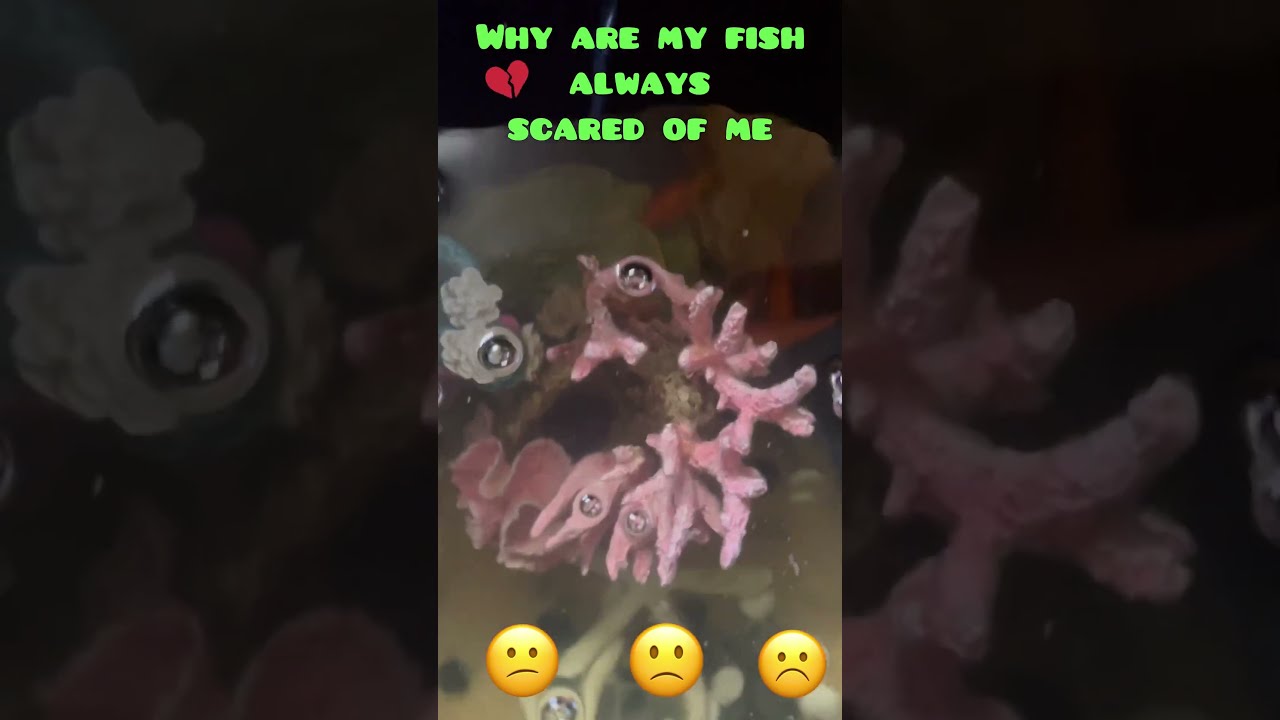The image appears to be a screenshot, likely taken from a social media platform such as TikTok or Instagram Live. It features a central piece of pink coral, possibly inside an aquarium, with scattered bubbles or fish eyes around it, although it's unclear if actual fish are present due to the poor image quality. The background showcases the main picture blown up and darkened on the left and right sides. At the top of the image, in green text, it reads "Why are my fish always scared of me" accompanied by a broken heart emoji. The bottom of the image displays three sad face emojis. The colors in the image include green, red, yellow, brown, pink, blue, black, white, and gray, and the overall composition suggests that it was taken for personal fun rather than professionally.